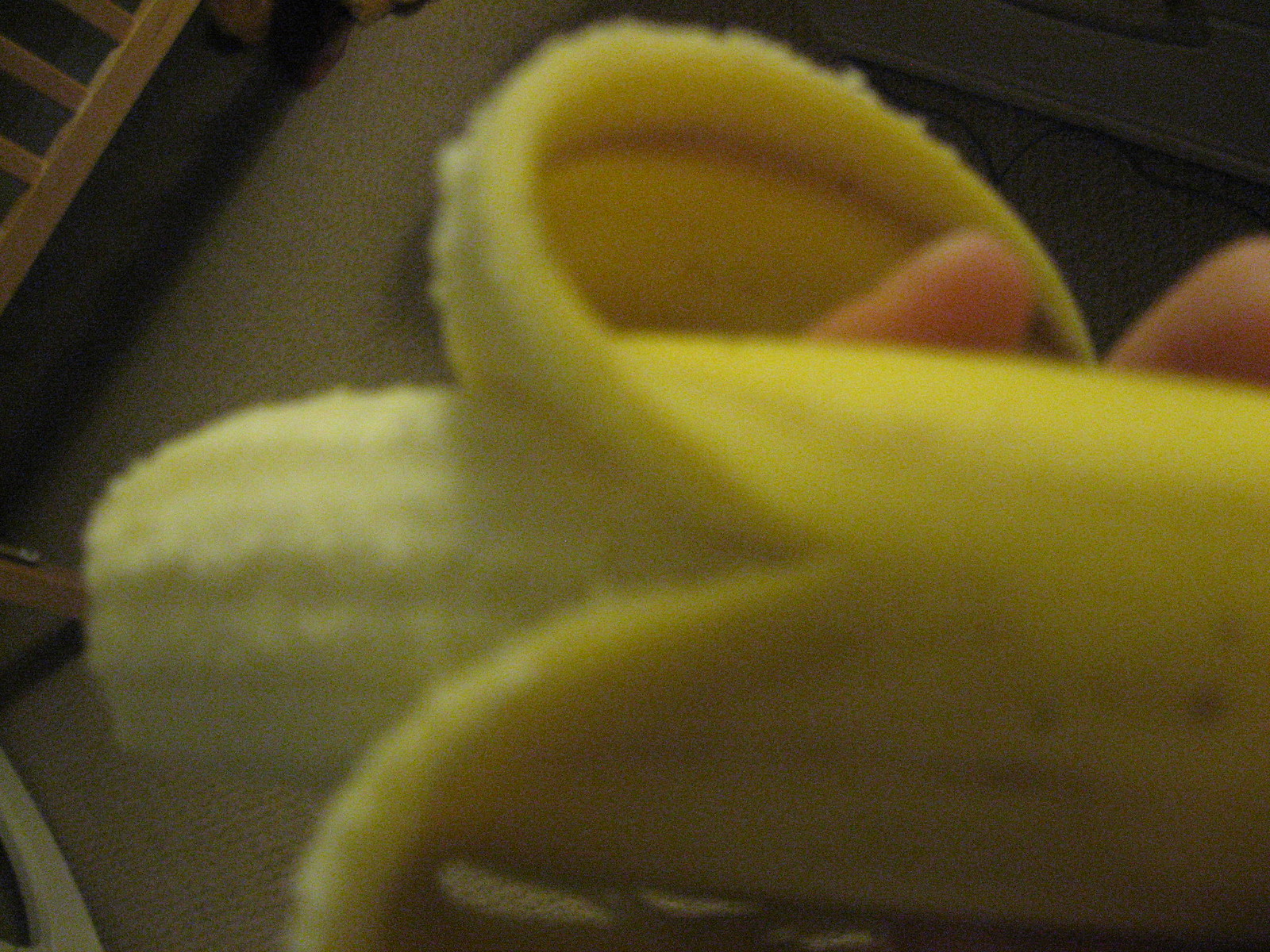A close-up, somewhat blurry photograph focuses on a half-peeled banana, revealing its split sides with one peel curled upwards and the other downwards, and a few inches of the banana exposed at the top. Two fingers are visible holding the banana from the back. The background features a brown Berber carpet, a wooden baby bed rail with visible legs, a partially seen teddy bear at the top of the image, a black cord extending across the carpet to the right, a flat platform with a central pedestal, and a plastic ring on the floor in the bottom left corner.